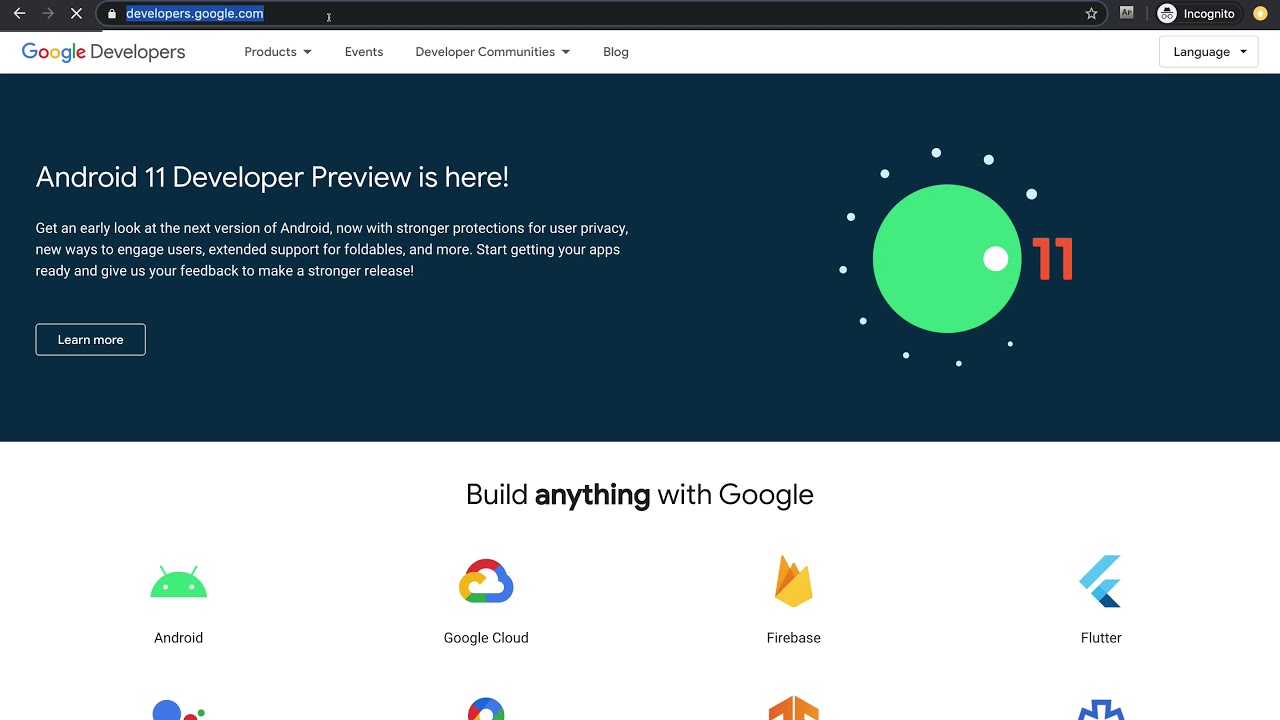This is a neatly formatted screenshot of a computer screen displaying the Google Developers website. The top of the screen features a black navigation bar running horizontally across the width of the page. On the upper left corner of this bar, there is a gray left-pointing arrow followed by a gray "X." The upper right corner contains various hard-to-see icons.

Beneath the black bar is a gray header that prominently reads "Google Developers," with "Google" colored in the traditional Google colors (blue, red, yellow, and green) and "Developers" in black. Adjacent to this header, there are several menu items: "Products" accompanied by a small black downward arrow, "Events," "Developer Communities" also with a small black downward arrow, "Blog," and finally, on the far right, a rectangular button that says "Language" with a down arrow beside it.

Below this header is a blue graphic rectangle. On the left side of this rectangle, in bold white text, it reads, "Android 11 Developer Preview is here." Below this headline, there are three lines of smaller white text, and approximately four lines further down, there is a white-outlined rectangle with the words "Learn More" written inside it in white.

To the right of this blue rectangle, there is a lime green circle. Located at what would be the three o'clock position on this circle is a smaller white circle, and just to its right, a bolded number "11." Surrounding the outer edge of the lime green circle near the designated hours are white dots symbolizing clock positions.

Intriguingly positioned below this section, against white space, is a header reading "Build Anything" in black text, with "Anything" boldly emphasized, followed by "with Google." Underneath, there are icons representing various Google developer tools and platforms. From left to right, the icons label "Android," "Google Cloud," "Freebase," "Flutter," and the tops of four additional icons are partially visible in the subsequent row.